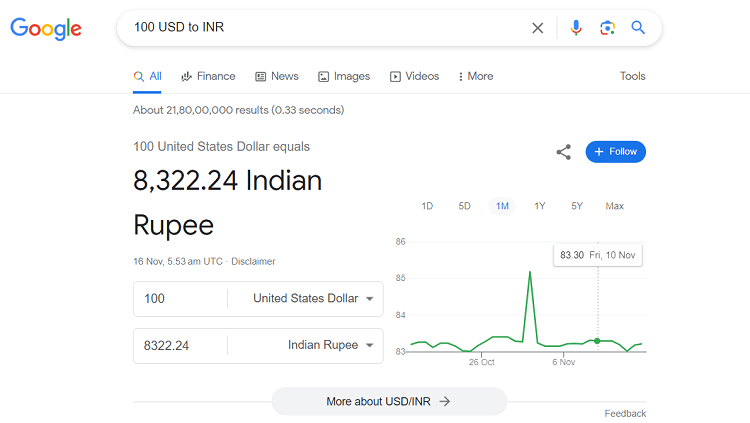The image is a detailed screenshot of a Google search result page displaying the conversion rate from US dollars (USD) to Indian Rupees (INR). The background of the page is white. At the top left, the Google logo is prominently featured in its signature colors: blue, red, yellow, blue, green, and red, respectively.

Within the Google search bar, the query "100 USD to INR" is typed in bold black text. Below the search bar, there are several menu options. The "All" tab is highlighted in blue with a magnifying glass icon next to it. To the right, other options include "Finance," "News," "Images," "Video," "More," and "Tools," all in dark gray lettering.

The search results indicate, in small gray font above the primary output, "100 USD equals." Below this, in large black font, "8,322.24 INR" is displayed. Beneath the primary conversion result, it is noted that there are approximately "21,800,000 results" found in "0.33 seconds."

The central portion of the screenshot showcases a graph illustrating the historical exchange rate of the Indian Rupee. The graph features a green line tracking the value over time, with a white rectangle at the point marked "83.30" the rate on Friday, 10 November, indicated by a gray dotted line extending from this marker. The x-axis of the graph spans from "26 October" on the left to "6 Nov" on the right.

To the left of the graph, there are further details converting the number of US dollars to Indian Rupees. Just above the graph, options for different time resolutions of the exchange rate are available: "1 day," "5 day," "1 month," "1 year," "5 year," and "max."

At the bottom of the image, in a rounded gray text box, there is an option reading "More about USD/INR" followed by a right-pointing arrow, indicating the availability of additional information. Towards the bottom right, the option for "Feedback" is listed in gray text.